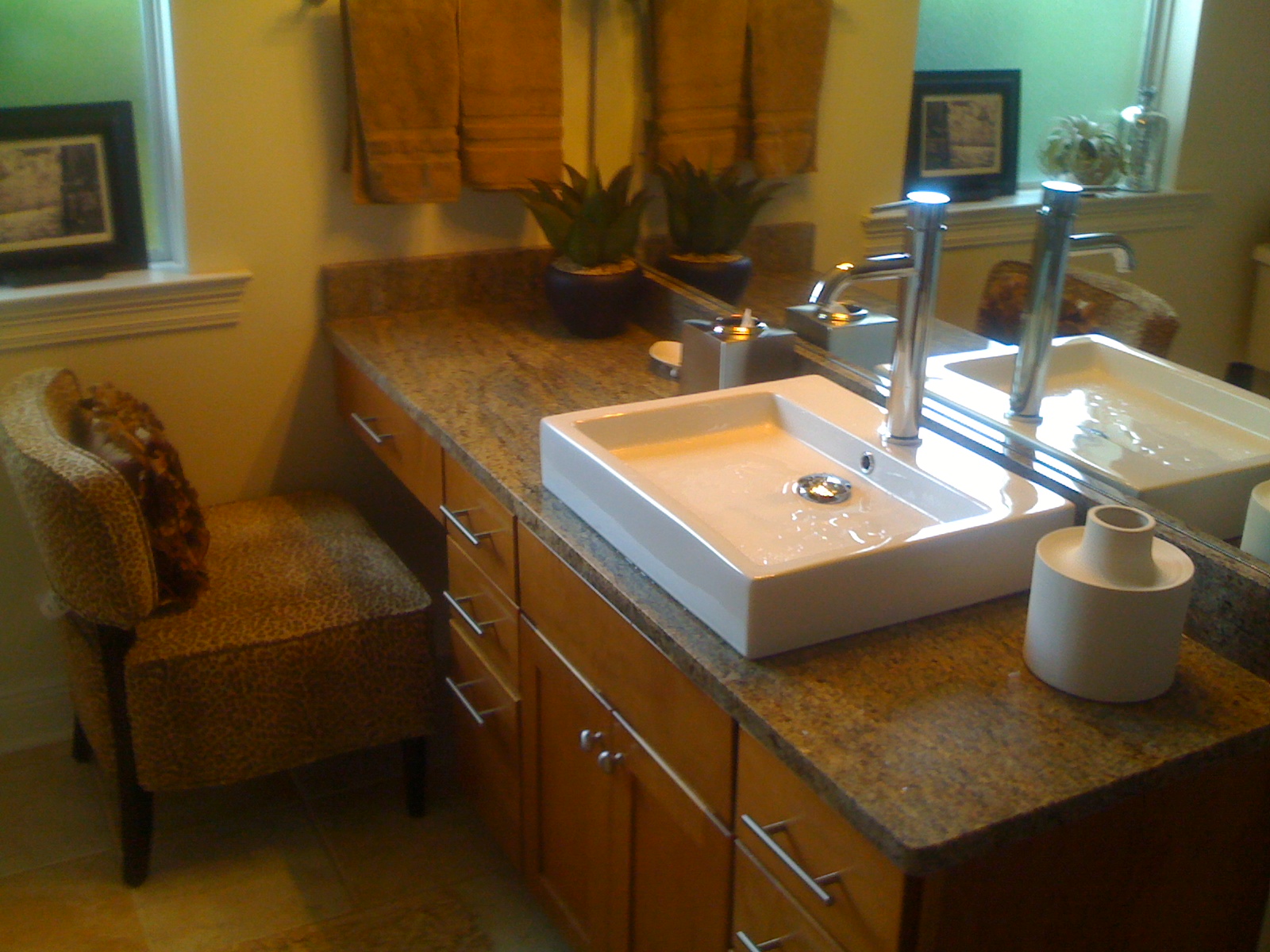A cozy and well-appointed bathroom is captured with several noteworthy elements. In the upper left corner, a window with a green shade partially drawn down allows minimal light. Perched on the window sill and leaning against the shade is a black-framed photograph or image, set in what appears to be a wooden frame. Adjacent to the window, a couple of reddish-brown hand towels hang neatly from a horizontal towel rack, giving a warm touch to the space. These towels are reflected in a mirror positioned immediately to their right, creating the illusion of four towels. Below the towels, a potted plant—potentially artificial—adds a splash of greenery and is situated on a brown mottled countertop, which features a range of shades from brown to tan. 

The centerpiece of the countertop is a shallow tray basin-like sink with some water in it, complemented by a sleek, stainless steel faucet that stands vertically with a horizontal spout directing leftward. The vanity below is wooden with modern stainless steel handles, blending functionality with style. To the left of this vanity, a low, padded chair is tucked almost up against the open space at the bottom, topped with a brown fuzzy pillow for added comfort. The entire scene is mirrored in a large mirror at the back of the vanity, enhancing the depth and reflective light in the room. The overall aesthetic is both warm and inviting, with a balance of natural elements and modern design.